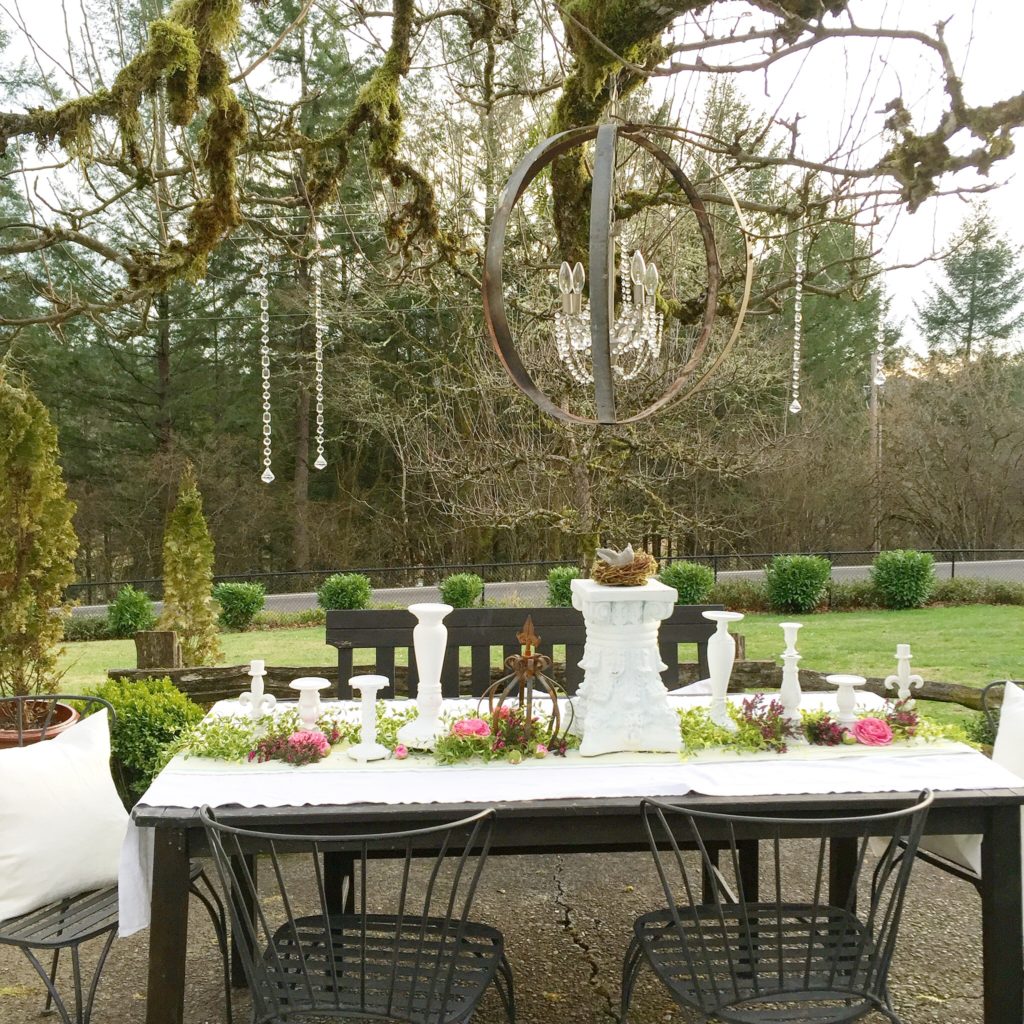This outdoor daytime photograph captures a picturesque patio area, perfect for a genteel gathering or a wedding reception. Dominating the foreground is a long table draped with a pristine white tablecloth, positioned horizontally from the right edge toward the left edge of the frame. The table is surrounded by metal chairs with wire backs, most notably featuring a white pillow on the chair to the left. One can spot a hint of a wooden bench running along the opposite side of the table.

Adorning the table are various white objects, including small and large candle holders and vases mixed with an array of flowers and leaves. In the center, there is a notable platform with a decorative nest, possibly housing a bird figure. To the left of this, a potted plant adds to the botanical theme. The objects are meticulously arranged, contributing to an elegant tabletop display.

In the background, a well-manicured lawn leads to a row of neatly trimmed shrubs lining a cement barrier, beyond which lies a road. Behind the road, a dense wooded area is visible, giving a sense of seclusion and tranquility. overhead, from the branches of a tree—partially visible in the frame—hangs an intriguing metal mobile surrounded by decorative chains and small jewel-like hangings. Some branches are festooned with moss, enhancing the rustic charm of the setting. The entire scene rests on a slightly cracked concrete surface, adding a touch of authenticity to this charming outdoor space.